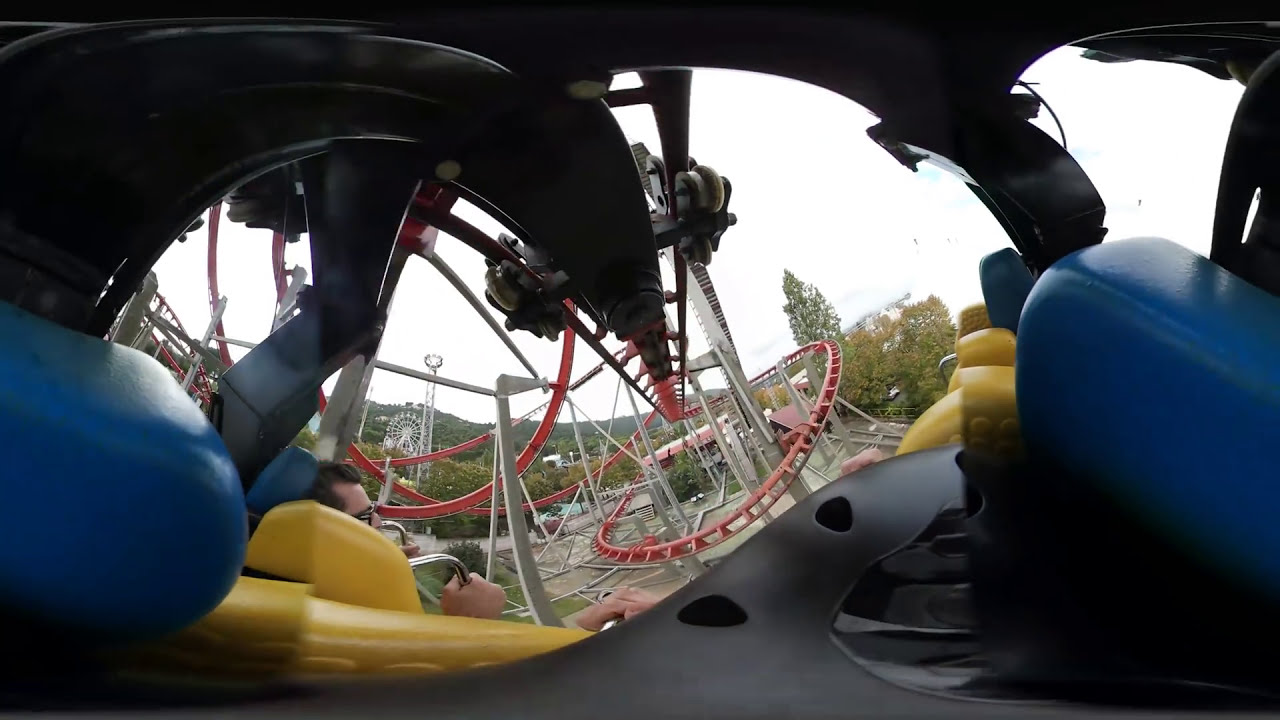The image captures the exhilarating experience of a high-intensity roller coaster ride, taken either from a rider's perspective or a camera onboard the ride. The roller coaster, characterized by its red tracks and white supports, features numerous sharp curves and turns. The riders, visible in the bottom left of the image, are strapped into yellow and blue seats, gripping stainless steel safety bars. One rider, likely a man wearing glasses, is seen clutching the bars by his chest. The backdrop reveals a sprawling amusement park with abundant trees, suggesting it is either late summer or early fall due to some yellowing foliage. Prominently in the background are additional park attractions, including a towering Ferris wheel and other tall structures. The sky above is clear yet somewhat blurry, indicating a bright day with diffused sunlight, possibly overcast. The overall color palette of the image includes splashes of red, yellow, blue, green, and metallic hues, vividly capturing the dynamic and vibrant environment of a bustling amusement park at midday.